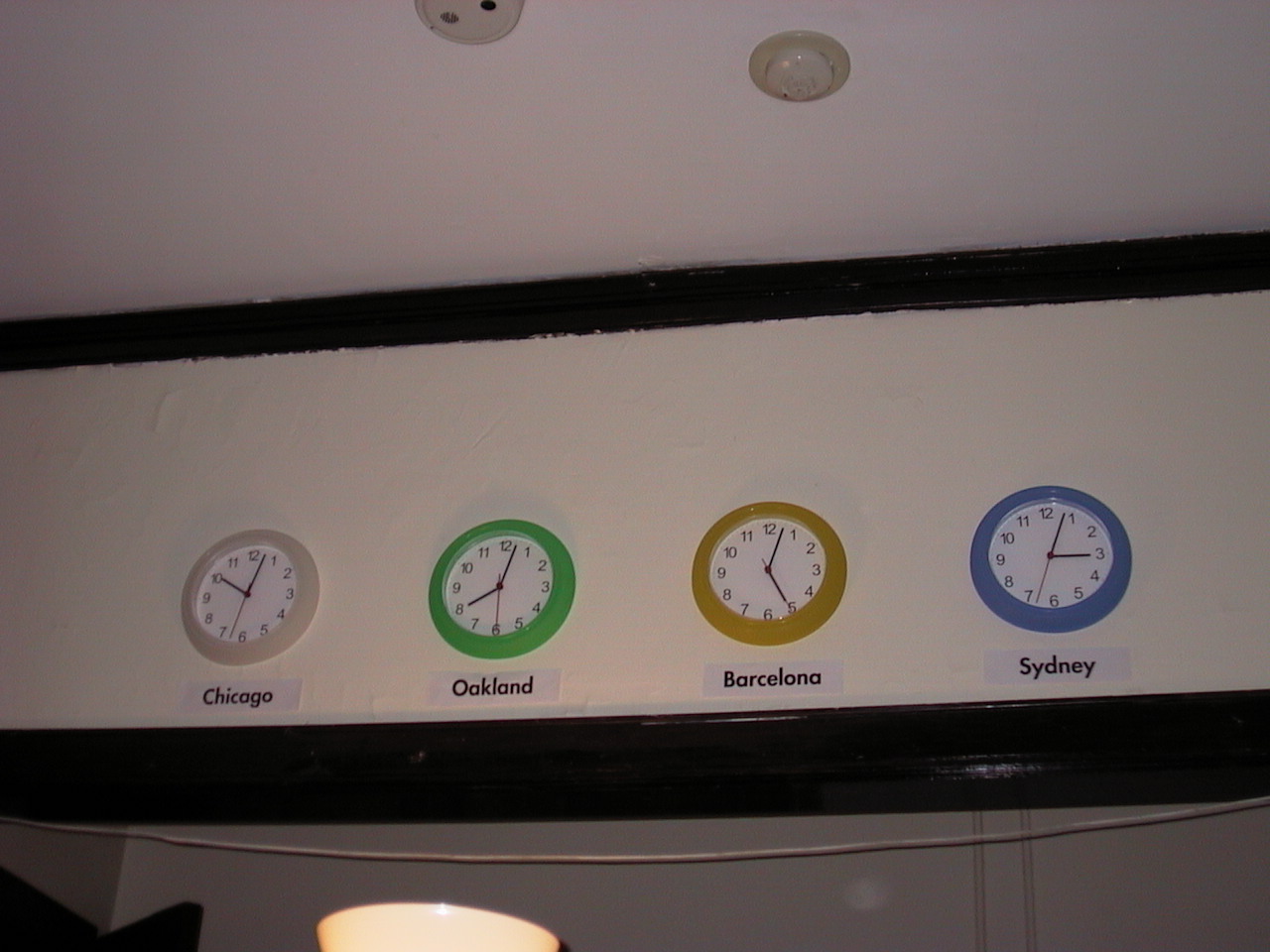The image is a detailed color photograph taken looking up at the top portion of a wall, which is predominantly white with black borders on both the top and bottom. The focus is on four round clocks mounted in a straight horizontal line along the white section of the wall. These clocks are framed in distinct colors: white for Chicago, green for Oakland, yellow for Barcelona, and blue for Sydney. Each clock shows the time for its respective city, with Chicago displaying 10:03, Oakland 8:03, Barcelona 5:03, and Sydney 3:03. The clock faces are white, enhancing the visibility of the times. Above the clocks, the ceiling can be seen featuring what appears to be a smoke alarm and a light fixture. The light socket is dark yellow, contrasting with the white ceiling. Below the clocks, a gray wall is visible, along with the top of a table lamp and a white cord hanging down.